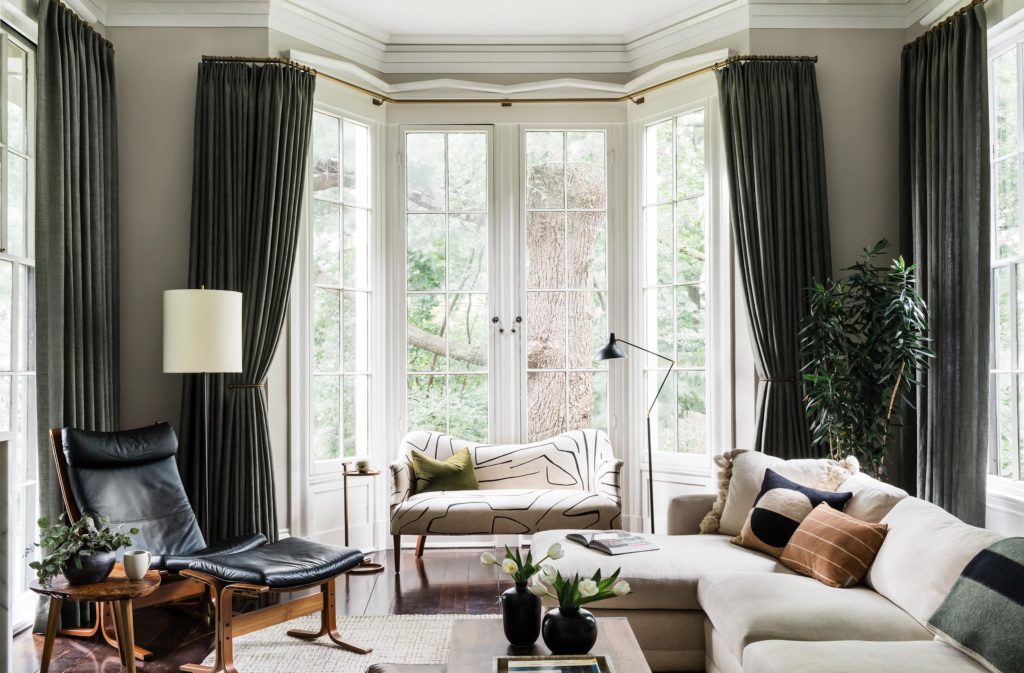This professionally photographed living room is a blend of modern elegance and comfort, bathed in natural light from expansive, floor-to-ceiling bay windows that span the room's three visible sides. The windows, adorned with dark gray and sage green curtains, frame a serene view of outdoor foliage. Centrally positioned in front of the bay windows is a small loveseat featuring a white cover with black abstract designs.

The left side of the room boasts a black leather lounge chair paired with a small table, which holds a leafy green plant and a coffee mug, while a tall reading lamp illuminates the corner. A stylish cream-colored sectional on the left is adorned with an array of pillows in black, white, and brown. A large coffee table in front of the sectional displays two black vases filled with white roses.

On the right side, a white couch, accented with three plush throw pillows, has an open book resting on its seat. Nearby stands a tall, vibrant plant, adding a touch of nature to the room's sophisticated decor. The room is meticulously decorated with post-modern furniture, additional lamps, and accent pieces, creating a cohesive and inviting living space.